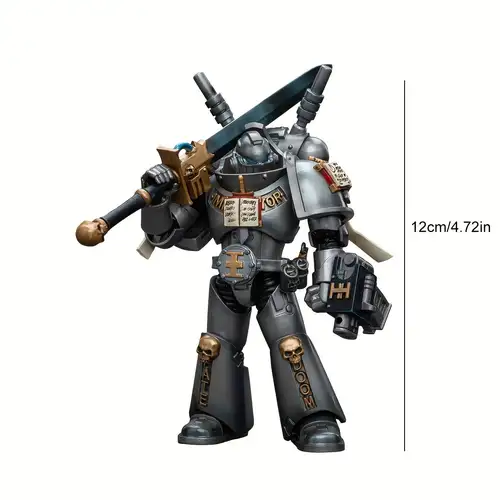This image showcases a detailed action figure styled after a Power Ranger-type character, standing still in a dynamic pose. The character is heavily armored with a puffy, plastic-like suit that obscures his head, which appears sunken into the neck of his elaborate armor. He wields a massive sword over his shoulder and holds a gun, probably part of a machine gun, in his other hand. The armor features various intricate designs, including skulls on his knee guards and the word "Doom" inscribed on one of his shin guards. The figure has additional weaponry or essential gear protruding from his back, possibly including a jetpack, indicating his ability to fly. His pants are reinforced with shields covering the thighs and shins, and he wears black shoes. His chest armor displays an artistic motif resembling an open book with a sword. The figure is a small statue, measuring 12 centimeters (4.72 inches) in height, as indicated by the vertical measurement line on the side of the display.